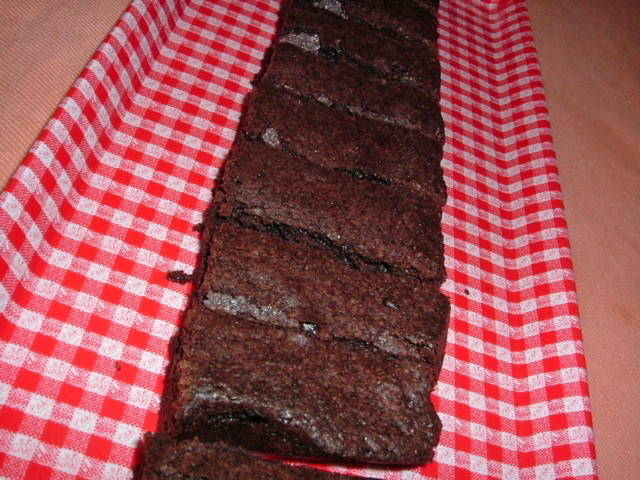This image captures a row of large chocolate brownies arranged on a red and white checkered tray, viewed from a bird's-eye perspective. The tray is positioned with its long sides running from the foreground to the background, while the brownies' long sides align horizontally across the image. There are 8 clearly visible brownies, with a possible 9th peeking out from the bottom edge, extending towards the top of the image in a line. The brownies appear darker towards the background and lighter in the foreground, suggesting a gradient in lighting from brighter at the front to darker as it recedes. The entire setup rests upon a light dirty pink tablecloth, adding a subtle warmth to the scene. Chocolate chips are visible in the brownies, possibly indicating a commercial setting due to the quantity and presentation.